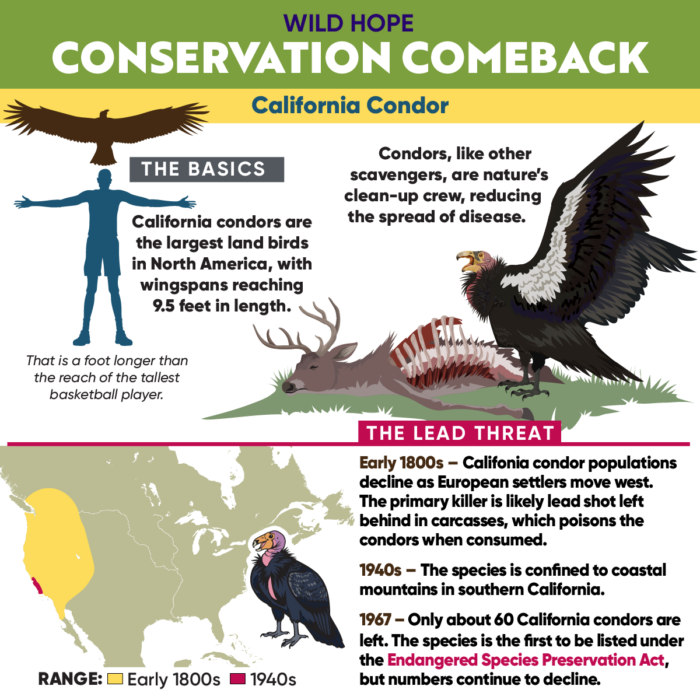The digitally created graphic titled "Wild Hope Conservation Comeback" focuses on the California Condor, highlighting their significance and the challenges they face. At the top, a green rectangle with text "Conservation Comeback" is followed by a yellow rectangle labeled "California Condor." Below, a graphic compares the wingspan of the California Condor, the largest land bird in North America with wingspans reaching 9.5 feet, to the arm span of a person, noting it is a foot longer than the reach of the tallest basketball player. An illustrated image to the right shows the condor feeding on a cartoon deer carcass, emphasizing that condors, like other scavengers, serve as nature’s cleanup crew, reducing the spread of disease. The bottom section, outlined by a red line and titled "The Lead Threat," narrates the decline of the species: from population reductions in the early 1800s due to European settlers, to being confined to Southern California's coastal mountains by the 1940s. By 1967, only about 60 condors remained, leading to their listing under the Endangered Species Preservation Act, although numbers continued to decline.